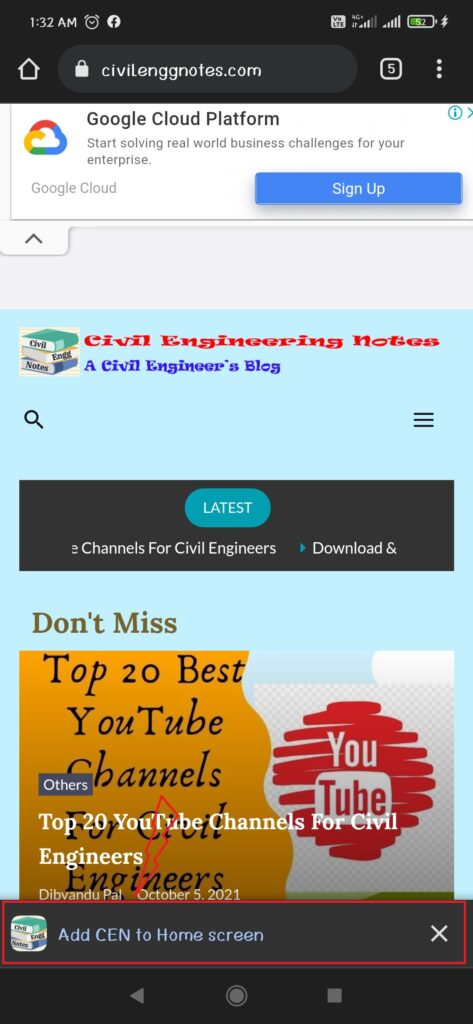A screenshot captured from the mobile site of civilengineernotes.com. The status indicators at the top display the time as 1:32 AM, accompanied by icons for an alarm clock, Facebook, LTE, and signal strengths showing 3 out of 5 bars for one type of service and 5 out of 5 bars for another. The device's battery is at 52% and charging, indicated by a green icon. 

The navigation bar below shows options such as Home and a lock icon, with civilengineernotes.com in the search box. A counter shows 5 open tabs, and a hamburger menu is present. The main screen features a banner for Google Cloud Platform with the colorful Google Cloud icon and a promotional line: "Start solving real-world business challenges for your enterprise." Below are buttons for Google Cloud and a signup link in blue with white text.

Further down, the site name "civilengineernotes.com" is displayed in a playful font, transitioning from red at the top to blue at the bottom, accompanied by a stack of books. The "Latest" section is highlighted in a teal box with white text, guiding users to content like channels for civil engineers. Another gray-black box features text promoting the "Top 20 Best YouTube Channels for Civil Engineers" with a YouTube icon.

Additionally, there's an option to add CEN to the home screen, which is situated above a mini box, likely a compact content preview or a call to action.